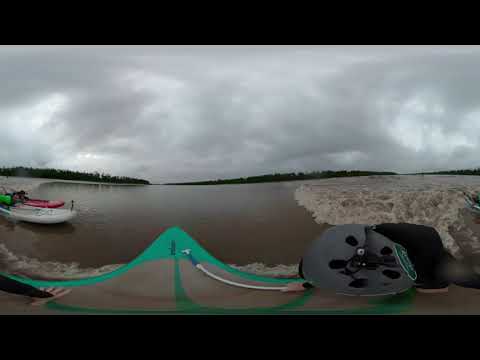The image is an outdoor scene with a fisheye lens perspective, featuring a lake under a gray, overcast sky occupying the top 40% of the picture. The distant tree line is visible along the horizon, forming a natural frame. To the left side, there are two small, motorized dinghies—the one at the back is red, while the one in the front is white. They appear to be made of plastic or rubber and are partially in the murky, brownish lake water. A green object is sitting in one of the boats, possibly the foreground boat, which might be a kayak or a raft. On the right side of the image, a sandy shore takes up about 30% of the frame. At the bottom part of the picture, there is a greenish netting lying on the ground, and a grayish, circular object that might be an umbrella or other indistinguishable equipment. The overall scene has an overcast and somewhat serene atmosphere, suggesting a calm day by a small lake.